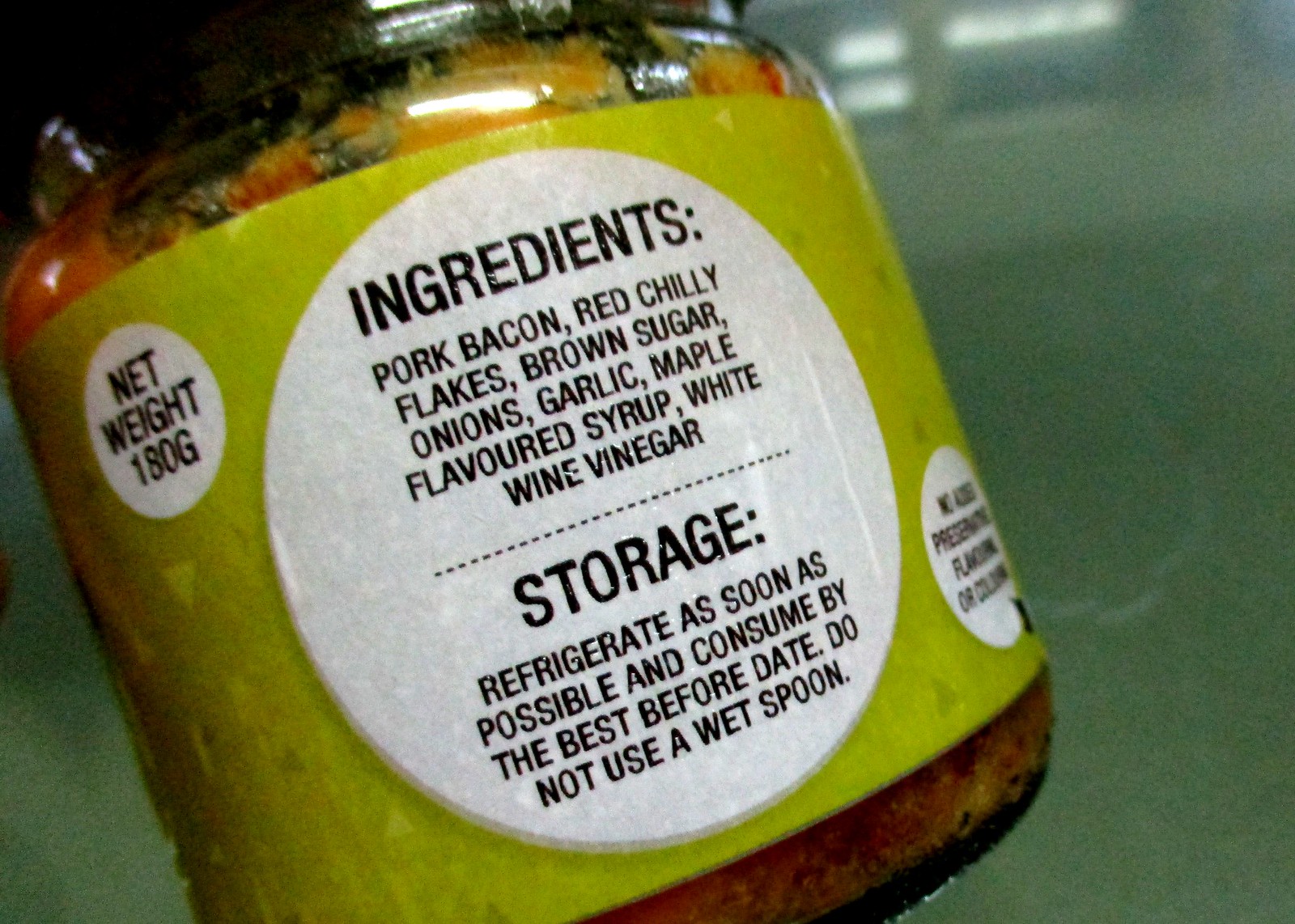This image is a detailed color photograph of a small glass food jar adorned with a green and white label. The label features three distinctive white circles with important information. The top left circle, smaller in size, specifies the net weight as 180 grams. The prominent central circle in black text lists the detailed ingredients, including pork bacon, red chili flakes (interestingly misspelled as "chilly"), brown sugar, onions, garlic, maple flavored syrup, and white wine vinegar. This section also includes storage instructions: "Refrigerate as soon as possible and consume by the best before date. Do not use a wet spoon." Another smaller circle on the label specifies that there are no added preservatives, flavors, or colors. The substance inside the jar appears to be a mix of these listed ingredients.